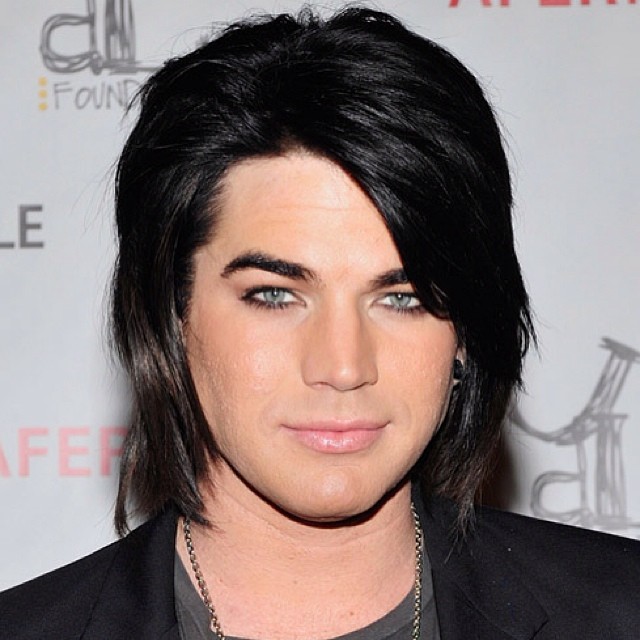The photograph captures a headshot of a man from his upper shoulders upwards, dressed in a black business coat and a gray shirt, accentuated with a silver chain necklace. His shoulder-length black hair frames his face, which features black eyeliner around his striking gray eyes, giving him a youthful yet mature appearance, suggesting he might be in his 40s. His ears are adorned with large black gauges in the lobes. The background is white, adorned with multiple logos mostly obscured by the man's head, with a partial readable logo appearing to be the letter "D" with the word "found" beneath it. The man's expression is slightly smirking, looking directly into the camera, adding a touch of charisma to his look.